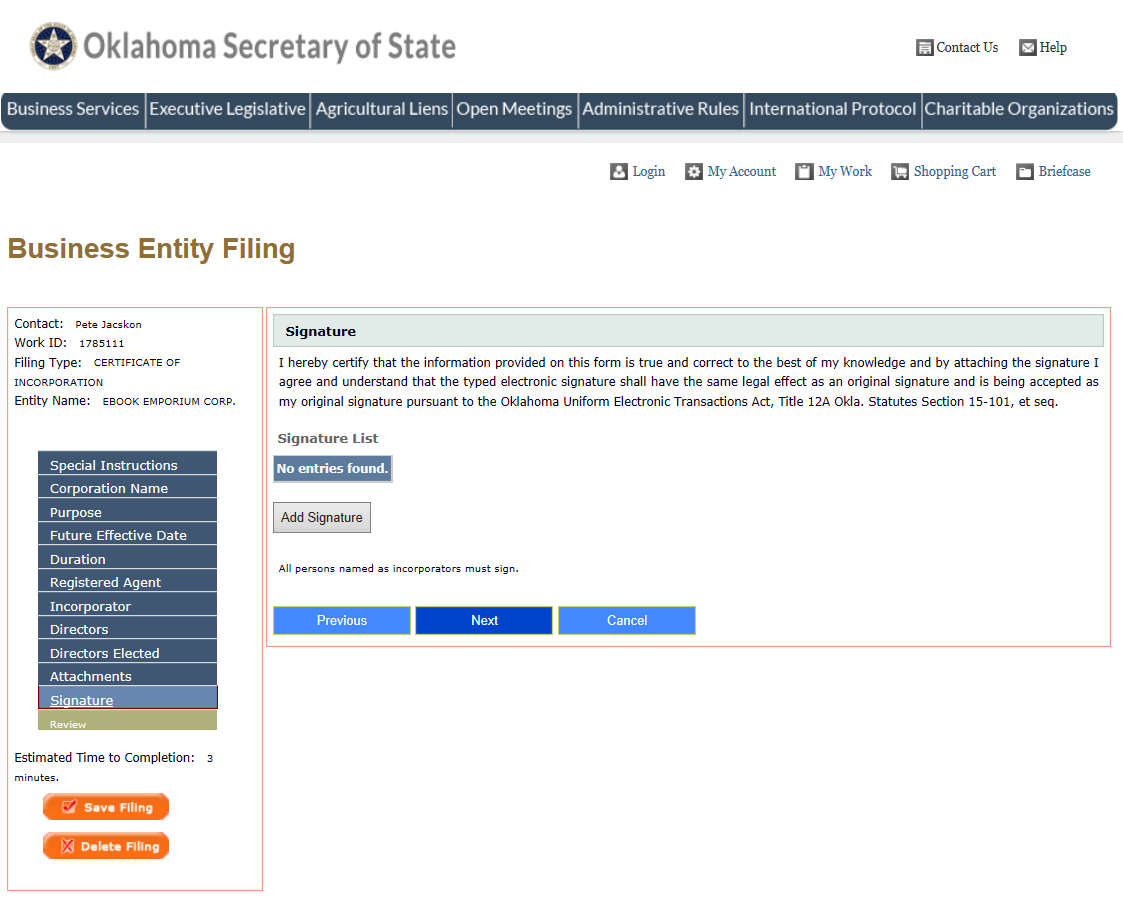The image depicts a screenshot of a website titled "Oklahoma State" prominently at the top. The main section of the page is labeled "Business Entity Filing." Centrally positioned on the webpage is a section marked "Signature," followed by a certification statement. The text reads: "I hereby certify that the information provided on this form is true and correct to the best of my knowledge, and by attaching the signature, I agree and understand that the typed electronic signature shall have the same legal effect as an original signature and is being accepted as my original signature pursuant to the Oklahoma Uniform Electronic Transmissions Act, Title 12A, Oklahoma Statute Section 15-101 et seq."